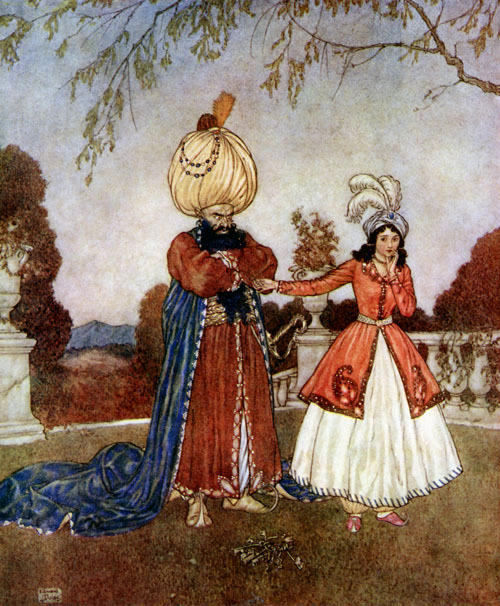This vertically aligned rectangular artwork captures a poignant outdoor scene that appears to be hand-painted. The setting is a richly detailed garden with a grassy surface and a stone wall, possibly a marbled fence, behind the characters. At the top of the composition, green leaves dangle from thin brown tree branches, set against a sky of blue, brown, gray, and white hues. 

In the center, we see two elegantly dressed figures. To the right, a woman in a long white dress and a red jacket that extends to her knees stands with her left hand on her chin. She wears pink shoes and a fancy hat adorned with three white feathers and blue accents. The woman reaches out with her right hand towards a man beside her. 

The man, portrayed with an air of regality, stands with his arms crossed, exuding a sense of displeasure. He has a large black beard and wears an ornate gold headdress adorned with jewels, resembling a sultan. His attire includes a flowing blue cape, a tan and ornately decorated robe, and a blue and gold belt around his waist. He stands firmly in a grassy area. 

In the background, there are outlines of trees and shrubs, with a stone pillar visible on the left and distant mountains under a gray sky. The detailed scene, full of intense colors such as green, red, brown, light blue, white, black, pink, orange, and tan, evokes a sense of historical narrative and emotional tension between the figures.